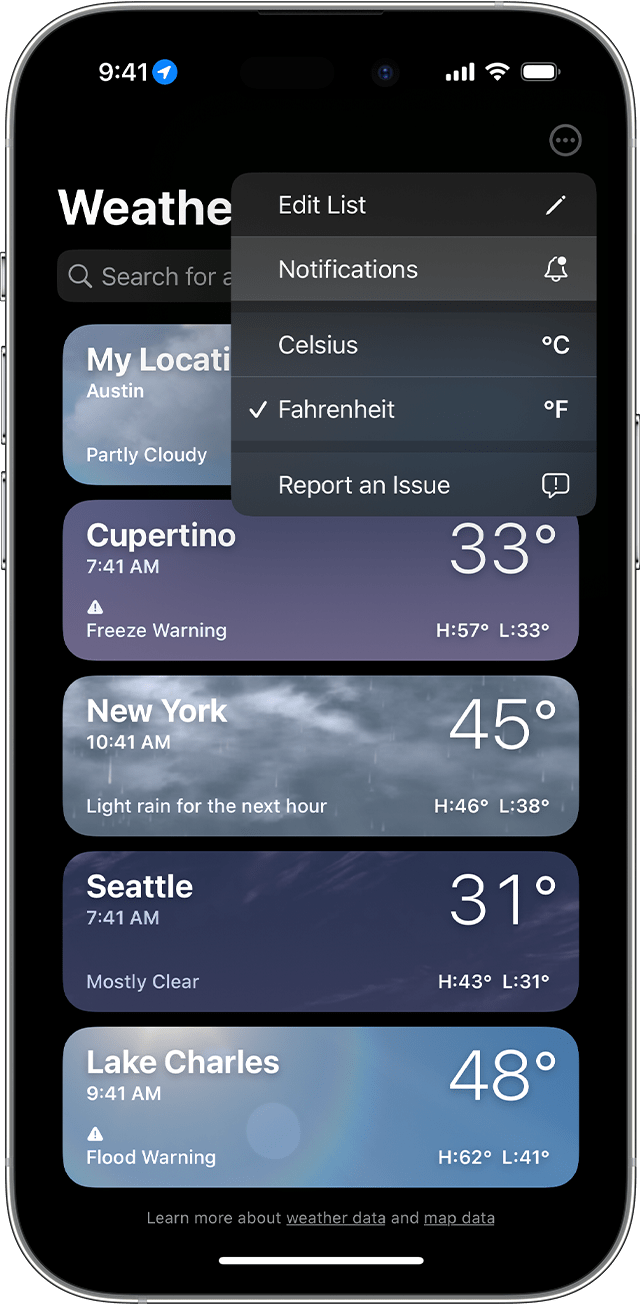The image displays a variety of weather data and notifications from multiple locations. 

At the top, the time in Cupertino is shown as 7:41 a.m., with a partly cloudy condition and a temperature of 30 degrees Celsius (equivalent to a high of 57 degrees Fahrenheit). 

In New York, it is currently 10:41 a.m., featuring a breeze warning with a temperature of 30 degrees Fahrenheit.

Seattle shows a time of 7:40 a.m., with mostly clear skies and a temperature range of 31 degrees Fahrenheit to a high of 43 degrees Fahrenheit. 

Lake Charles displays a time of 8:41 a.m., with a temperature of 40 degrees Fahrenheit, and a range from a high of 60 degrees Fahrenheit to a low of 41 degrees Fahrenheit.

Additionally, the image contains several rounded-corner rectangles that symbolize weather icons, depicting various conditions such as clouds and lightning. The user settings indicate an option to switch between Celsius and Fahrenheit units and include an interface for editing weather notifications.